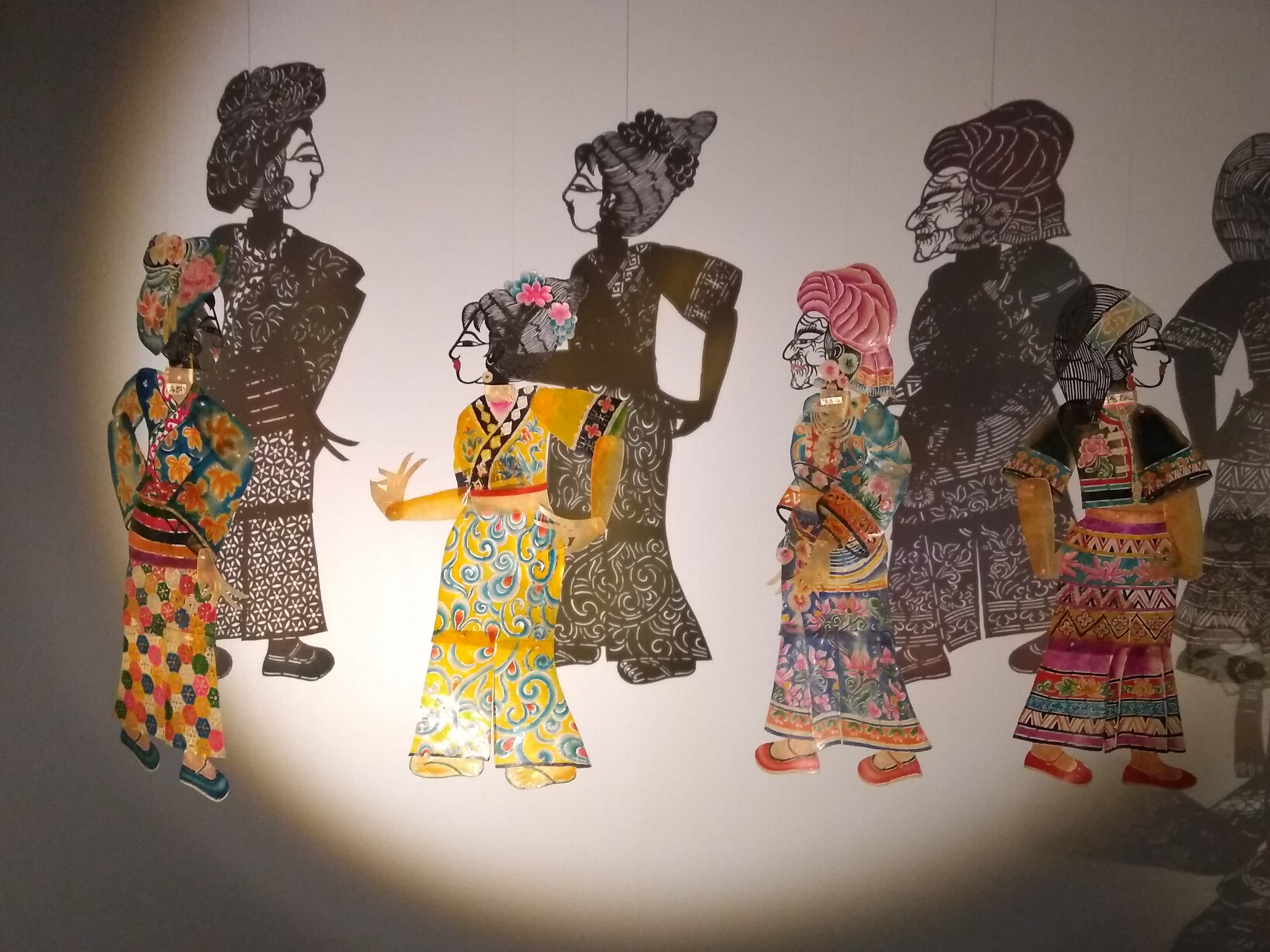The image features a detailed and ornate depiction of four women in traditional Japanese attire, rendered in a handmade drawing or painting style that incorporates both color and shadow. The central figures are four young women or children dressed in vibrant, multi-colored robes with decorative headpieces and traditional Japanese makeup, reminiscent of geishas. These paper cutouts are suspended, and a central light source casts their coordinated shadows on the wall behind them, presenting a dual-layer effect.

In the brightly lit center, the young woman on the far left wears a floral arrangement and faces toward the right. Second from the left, another young woman clad in yellow walks towards the first woman, while behind her stands an older, stern-looking woman dressed in a pink shawl and a floral dress. The rightmost figure features a young woman in a black top and a colorful, patterned skirt, facing left. 

The background shadows enhance the scene, featuring larger, darker silhouettes of the women, giving the image a striking depth. The contrast between the colored cutouts and their monochromatic shadows emphasizes the traditional Japanese elements, with flowers and colorful fabrics in their hair completing the intricate presentation. The use of light to cast prominent shadows around a darkened periphery amplifies the dramatic and cultural aesthetic of the artwork.